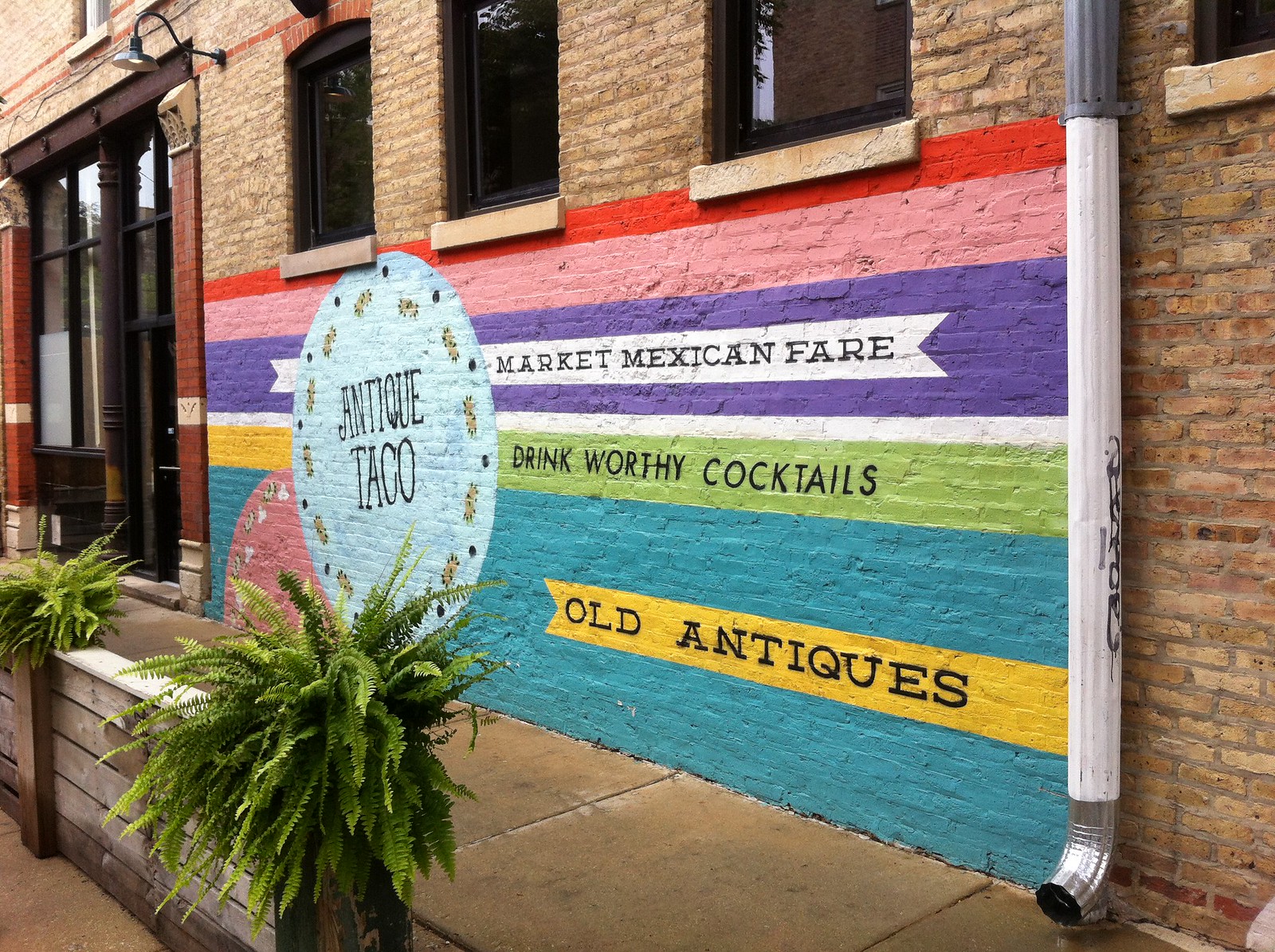The image depicts the exterior of a restaurant named "Antique Taco." The focal point is a large, painted, brick wall which has a worn, tan appearance in the unpainted areas. The painting covers the middle and bottom sections of the wall with colorful horizontal stripes. From top to bottom, the stripes are dark red, pink, purple, white, green, aqua blue, and yellow. 

At the center of the painted area is a large, light blue circle with the words "Antique Taco" in black text. Surrounding it, the purple stripe contains the phrases "Market" and "Mexican Fare" in black, intersected by a small white banner. The green stripe reads "Drink Worthy Cocktails" while the yellow stripe at the bottom declares "Old Antiques" in all capital letters.

Additional details include a partially painted white water spout on the right side and glass doors leading into the restaurant on the far left. The surrounding sidewalk is a brownish color, complementing the light brown of the unpainted brick.